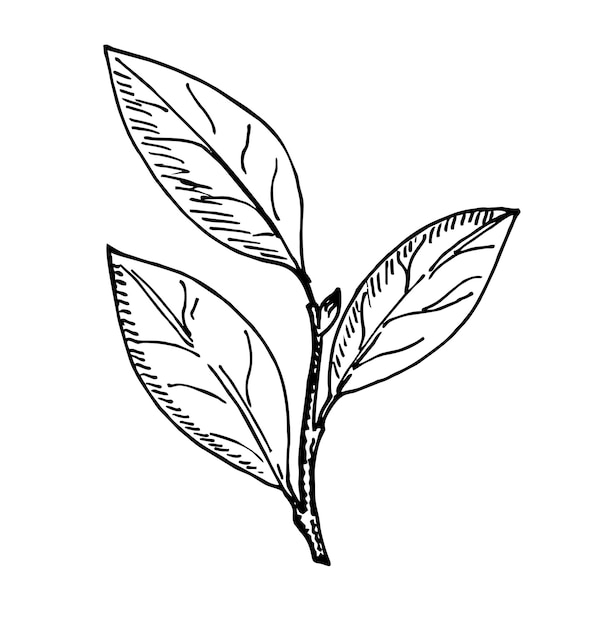This image is a detailed black and white line art illustration of a short plant stem with three prominently large, tapered leaves. The stem is depicted with a heavy dark line, while the leaves are outlined in finer lines and include hash marks for shadowing effects. The two leaves point upward towards the top left, and the third leaf points upward towards the top right, nestled between the first two. Near the top of the stem, there's a small bud, suggesting a new leaf or flower in the early stages of growth. Each leaf features a central vein with multiple small veins branching off symmetrically on both sides. The background is completely white, enhancing the floating effect of the illustration, which resembles artwork suited for a cartoon or a children's coloring book.